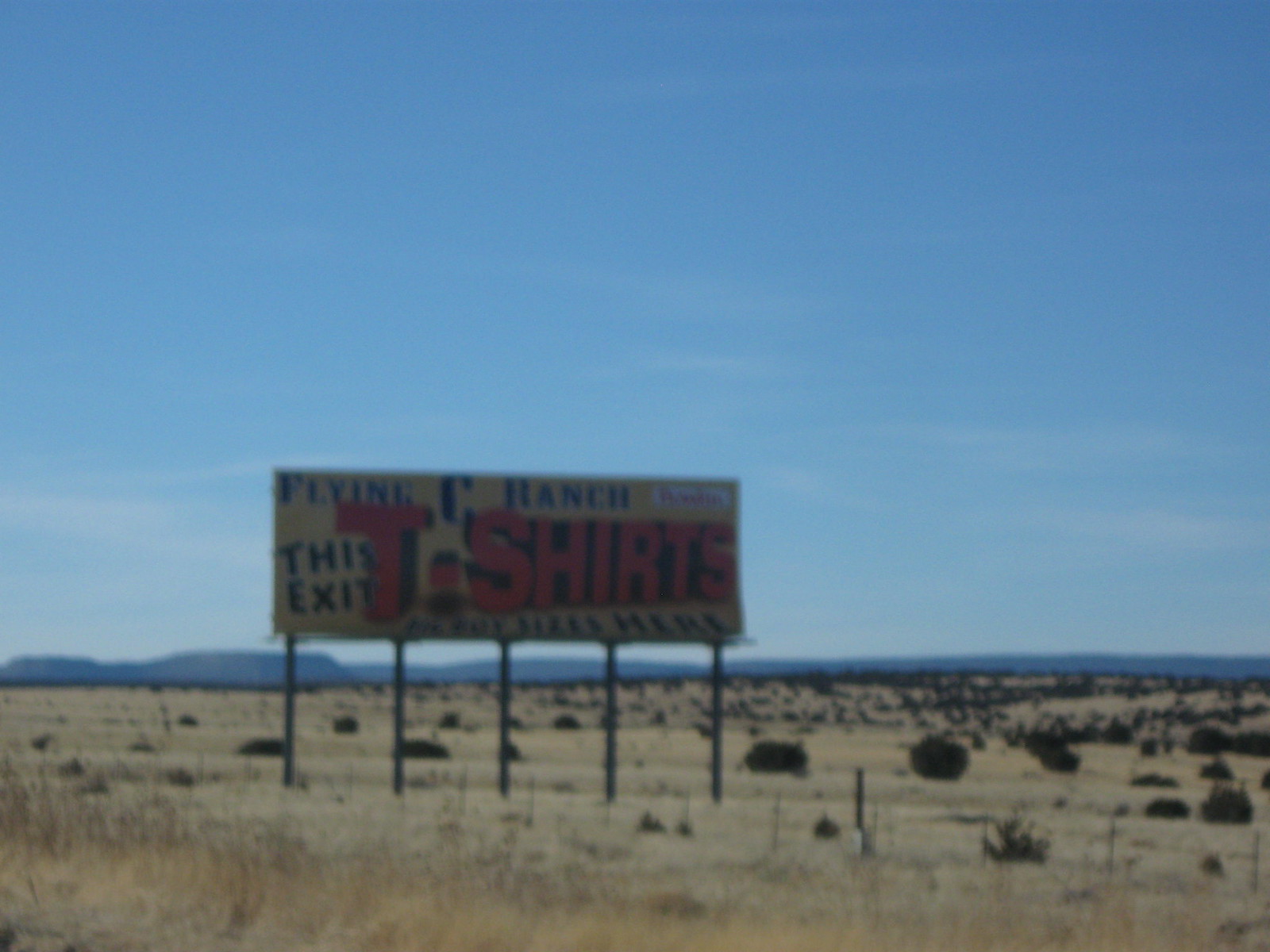The image depicts a low-quality, slightly blurry photo, likely taken with an older camera from a first-person viewpoint, potentially out of a car window on the road or roadside. The scene captures a short, somewhat medium to small yellow-brown billboard secured by five steel poles, situated in a sparse desert-like landscape characterized by tall grass, shrubs, and possibly tumbleweeds scattered throughout a paddock extending into the distance. In the background, a clear blue sky with some distant streaks of clouds stretches above the expansive, barren area.

Prominently displayed on the sign in bold red 3D letters is the word "T-SHIRTS," taking up a significant portion of the sign. Above this, in smaller blue text, reads "Flying Sea Ranch," with the phrase "this exit" placed to the left of "T-SHIRTS." There is additional smaller text at the bottom of the sign, but it is not legible due to the photo's quality. The overall scene suggests an advertisement for T-shirts available at the next exit, amidst a remote, roadside environment.